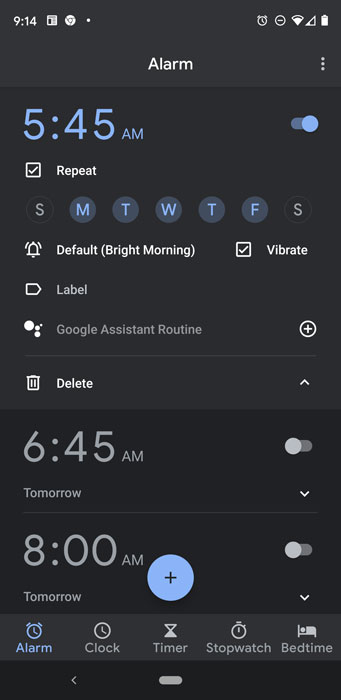This image features a smartphone's alarm settings page. At the top left, the time displays as 9:14. To the right, there are icons for a newspaper and Google Chrome, both in white, followed by a dot. On the far right, there is an alarm icon, a circular minus symbol, and a nearly full Wi-Fi signal indicator.

In the central part of the screen, a series of alarms are listed:
- The first alarm is set for 5:45 AM. To the right of this time is a dot.
  - Below this alarm, the word "Repeat" is followed by the weekdays: M-T-W-T-F-S.
  - The selected days highlighted are Monday, Tuesday, Wednesday, Thursday, and Friday.
  - Additional settings for this alarm include "Default," "Bright Morning," "Vibrate," "Label," and "Google System Routine."
  - The options "Default," "Bright Morning," and "Vibrate" are selected for this alarm.
- Below this, there is an option to "Delete" the alarm.
- Further down, there are additional alarms set for 6:45 AM and 8:00 AM.
- At the bottom, there is a plus sign (+) to add a new alarm.

At the very bottom row, there are options for "Alarm," "Clock," "Time," "Stopwatch," and "Bedtime." The "Alarm" option is highlighted in blue. Below this row, there is a red and black bar with a back arrow icon on the left and a gray bar in the middle.

None of the alarms are currently activated, as indicated by the absence of highlighted on/off toggles.